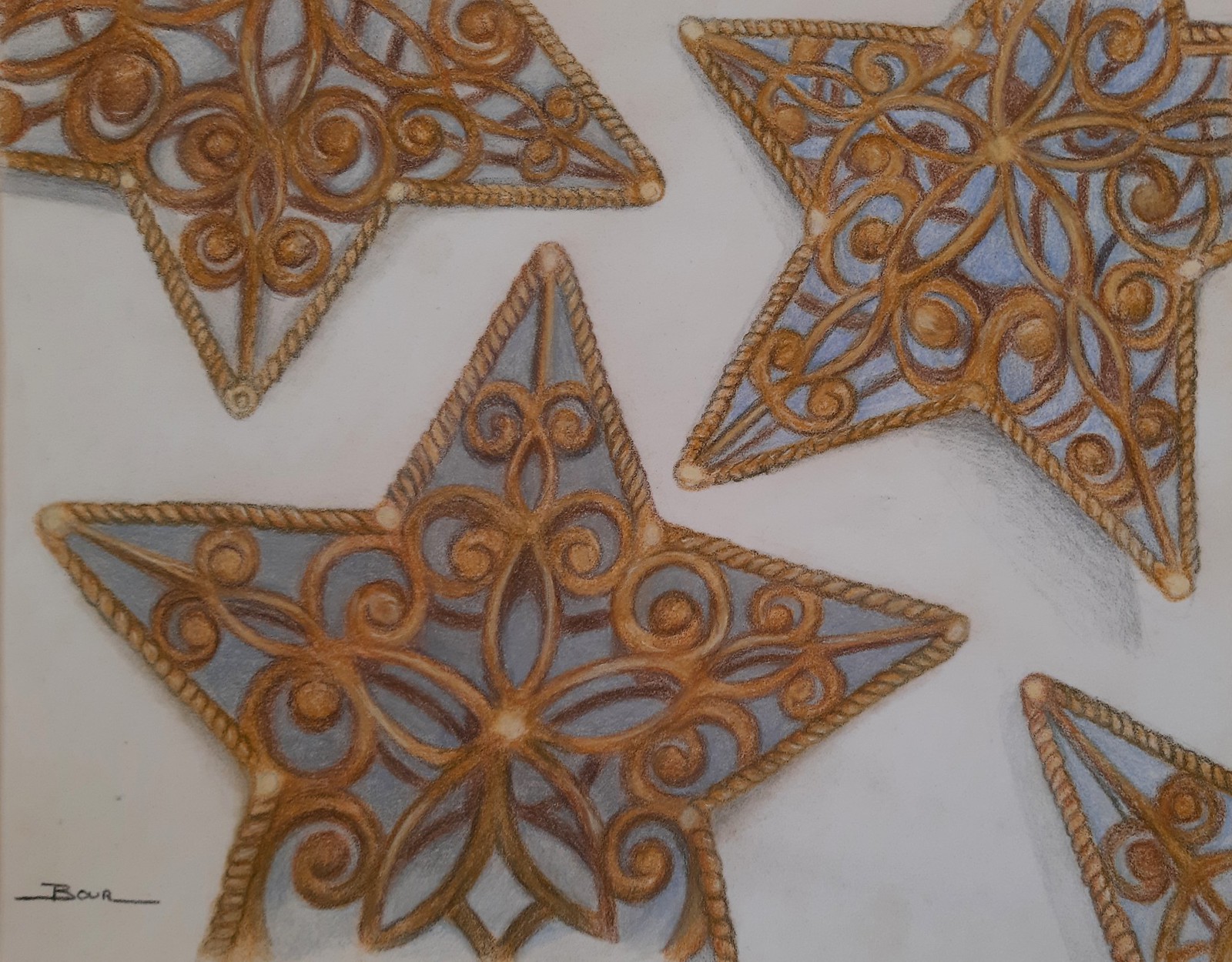This image is a detailed drawing on off-white paper, created using graphite and colored pencils. It portrays four three-dimensional stars, each crafted to look like metal with roped edges. The stars, which have a bronze and silver hue, feature intricate filigree and floral designs at their centers, with five-lobed flower-like patterns adding to their elegance. The spaces within the stars are filled with a light blue color, enhancing the metallic appearance. The positioning of the stars is varied: the upper right star casts a small shadow on the paper at the bottom of its point, adding depth, while the others are partially visible, creating a sense of overlap and continuity. A neat and masculine signature reading "B-O-U-R" is present in the lower left-hand corner, indicating the artist's name, Bauer.